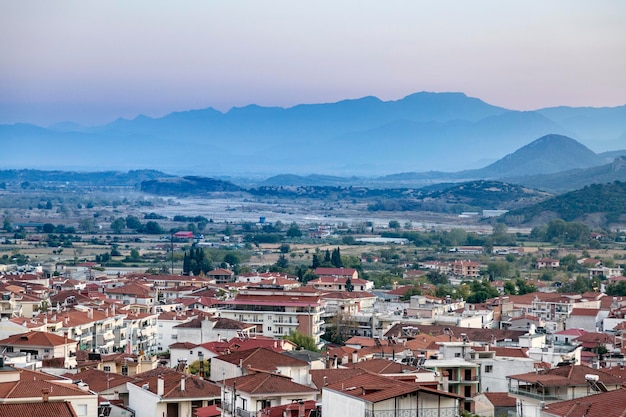This photograph captures an early morning, pre-sunrise view of a city or village nestled at the base of a mountain range. In the foreground, numerous cream-colored buildings with red-brown shingles form a tightly packed urban area. Power lines crisscross through the scene, adding to the bustling feel of the town. As the perspective stretches further back, the urban environment shifts to a more suburban landscape with scattered trees and more spaced-out houses, eventually merging into a barren countryside. The mid-ground features low-lying land with scattered vegetation before giving way to a light blue mountainous backdrop. The sky above is a purplish-gray, laden with clouds, completing the tranquil, atmospheric setting of the pre-dawn scene.